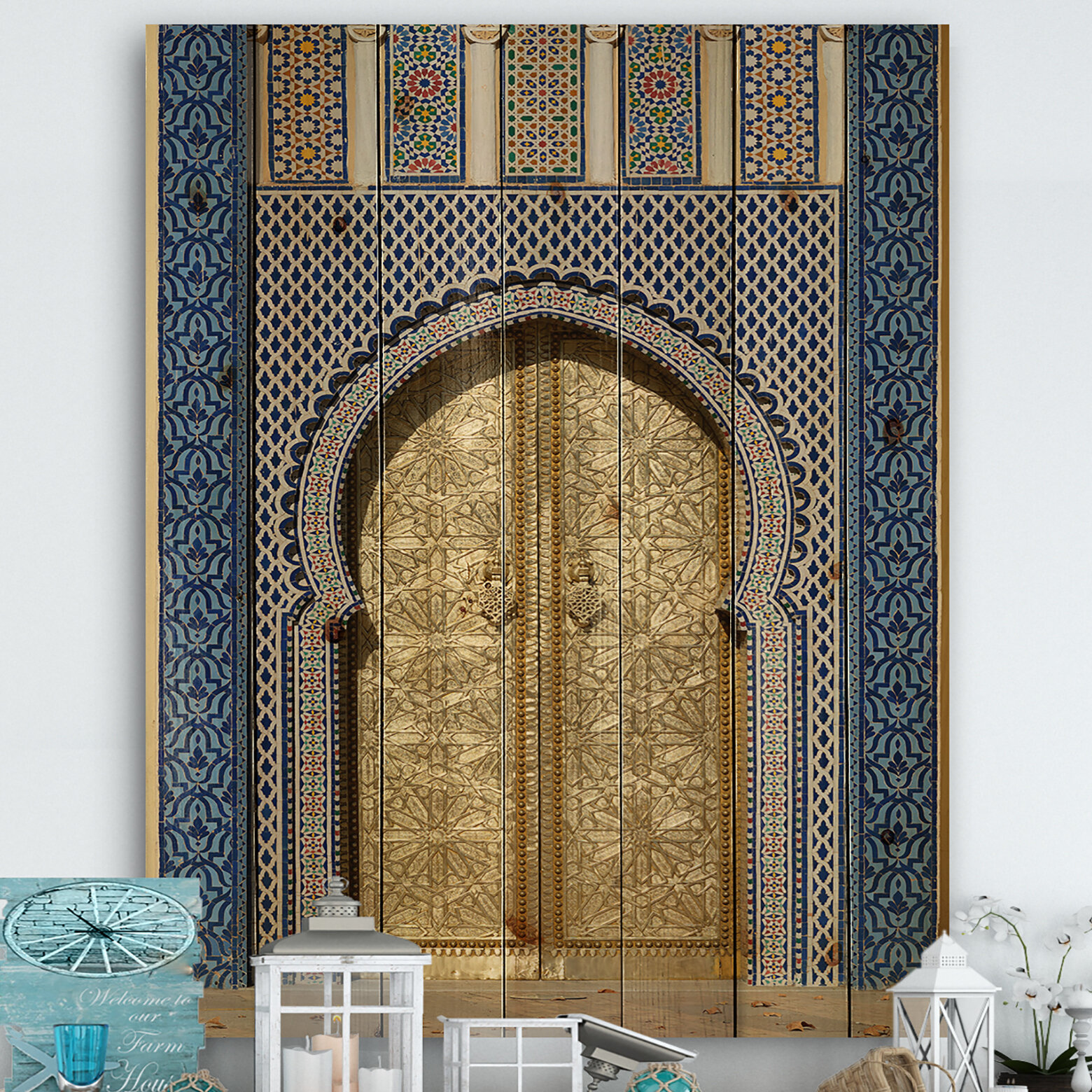This photograph features an incredibly ornate Persian-style door set against a white wall. The centerpiece is a pair of arched, golden double doors adorned with a spiralized radiant spoke pattern, flanked by sections of elaborate woodworking. The door is framed by intricate trim that mixes gold and teal-blue ornamentation, with designs resembling four Persian rugs sprawled across the top, and blue floral decorations on the sides. The base of the door has latticework elements, adding to the architectural grandeur.

In front of the door and somewhat cluttering the foreground, there are several white lanterns with candles, some upright and others tipped over. The fallen candles and an orchid plant in the lower right corner give the scene a slightly disordered look that contrasts with the meticulous design of the doorway. Additionally, various small objects, such as glass terrariums and a white wheel design on a blue box, are scattered at the bottom, contributing to the eclectic mix of items on the floor. This detailed and decorative doorway appears to be an artwork mounted on the wall, possibly a frameless canvas.